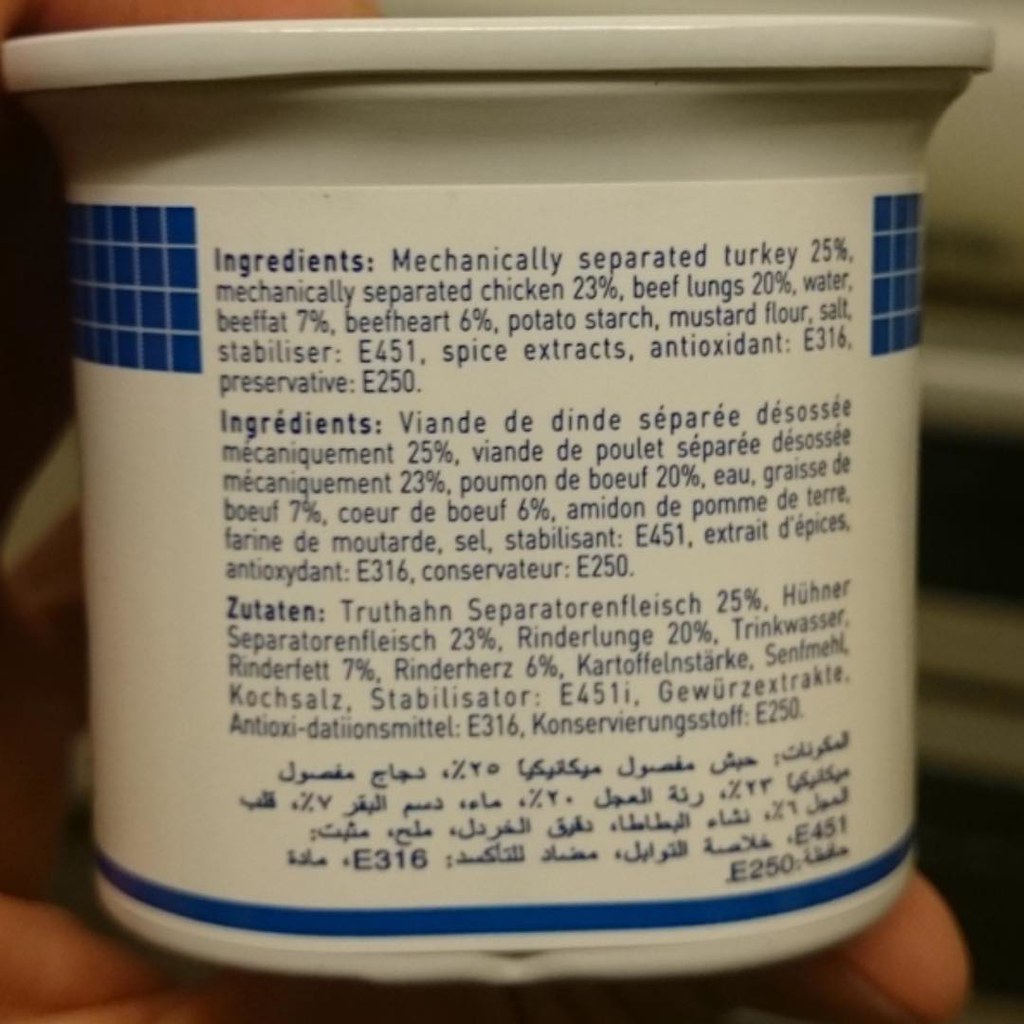This photograph captures a close-up of a can of food with a white plastic lid. The can itself is white with a detailed white and blue label. The label features blue font, prominently listing all the ingredients of the product. Notable ingredients include mechanically separated turkey (25%), mechanically separated chicken (23%), beef lungs (20%), water, beef fat (7%), beef heart (6%), potato starch, mustard flour, and various additives like salt stabilizer (E-451), spice extracts, antioxidant (E-316), and preservative (E-250). The bottom section of the label displays text in three different languages, indicating the global reach of the product. The can is being held up by a hand, which appears blurry, as does the background, emphasizing the contents and details of the label.